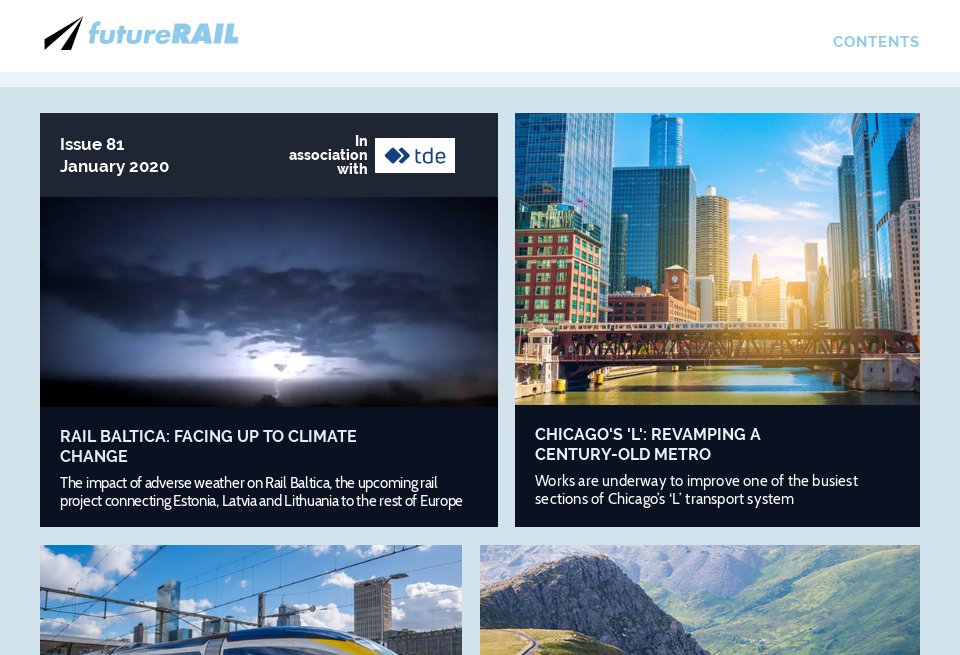This high-resolution screenshot is from the Future Rail magazine, easily identifiable by the brand logo positioned in the upper left-hand corner. Below the logo, the main section of the page features a large light blue square, which is segmented into four smaller boxes, each delineated for clarity.

In the top-left smaller box, the background is predominantly black, featuring a header with a black banner. This banner highlights "Issue 81" and "January 2020." Adjacent to this, a white banner prominently displays "In association with TDE," accompanied by two blue, 2D-styled square icons. Below this section, an evocative image captures a night scene with a dark sky and cloud cover. Just beneath the image, another black banner reads: "Rail Baltica: Facing Up to Climate Change - The impact of adverse weather on Rail Baltica, the upcoming rail project connecting Estonia, Latvia, and Lithuania to the rest of Europe."

In the top-right smaller box, the background features a sprawling cityscape dominated by towering business buildings, reminiscent of a bustling downtown area, possibly even Chicago. The accompanying text describes efforts in "Chicago's revamping of a century-old Metro," suggesting a focus on urban renewal and modernization.